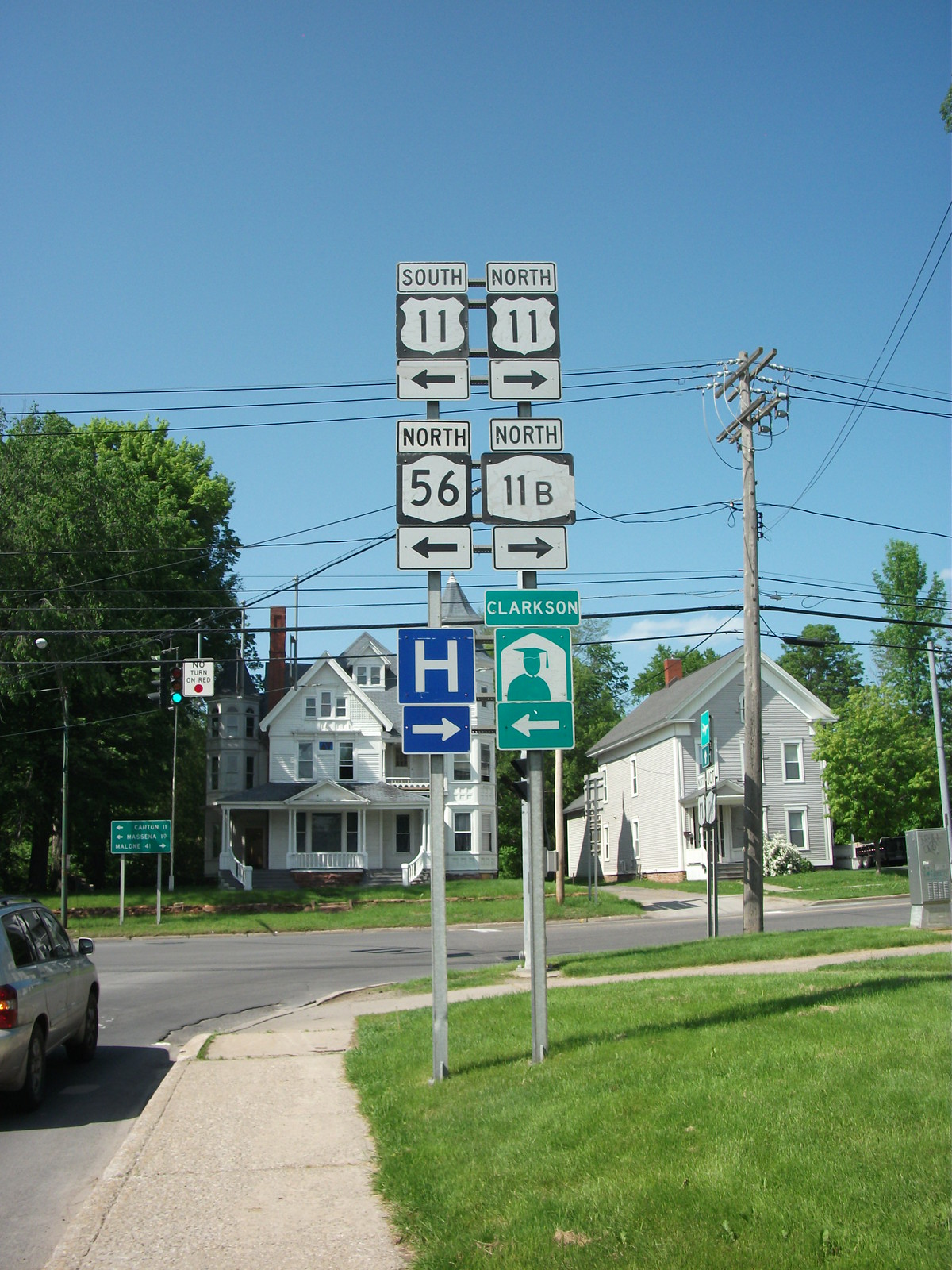This vibrant photograph, taken in portrait orientation, showcases a typical residential neighborhood street. At the center, a cluster of six street signs provides direction: at the top left, "South 11"; directly next to it, "North 11"; followed by "North 56"; and then "North 11B" beneath it. An "H" with an arrow pointing right and "Clarkson" with an arrow pointing left complete the array of signposts. 

Framing the signs are two white houses, one on either side, and a white car parked nearby. The scene is enriched with lush green grass and trees, indicative of a well-kept suburban area. The setting is bathed in the gentle light of a clear blue sky, adding to the peaceful ambiance of the neighborhood. A sidewalk runs alongside the street, inviting pedestrians to take a stroll through this tranquil locale.